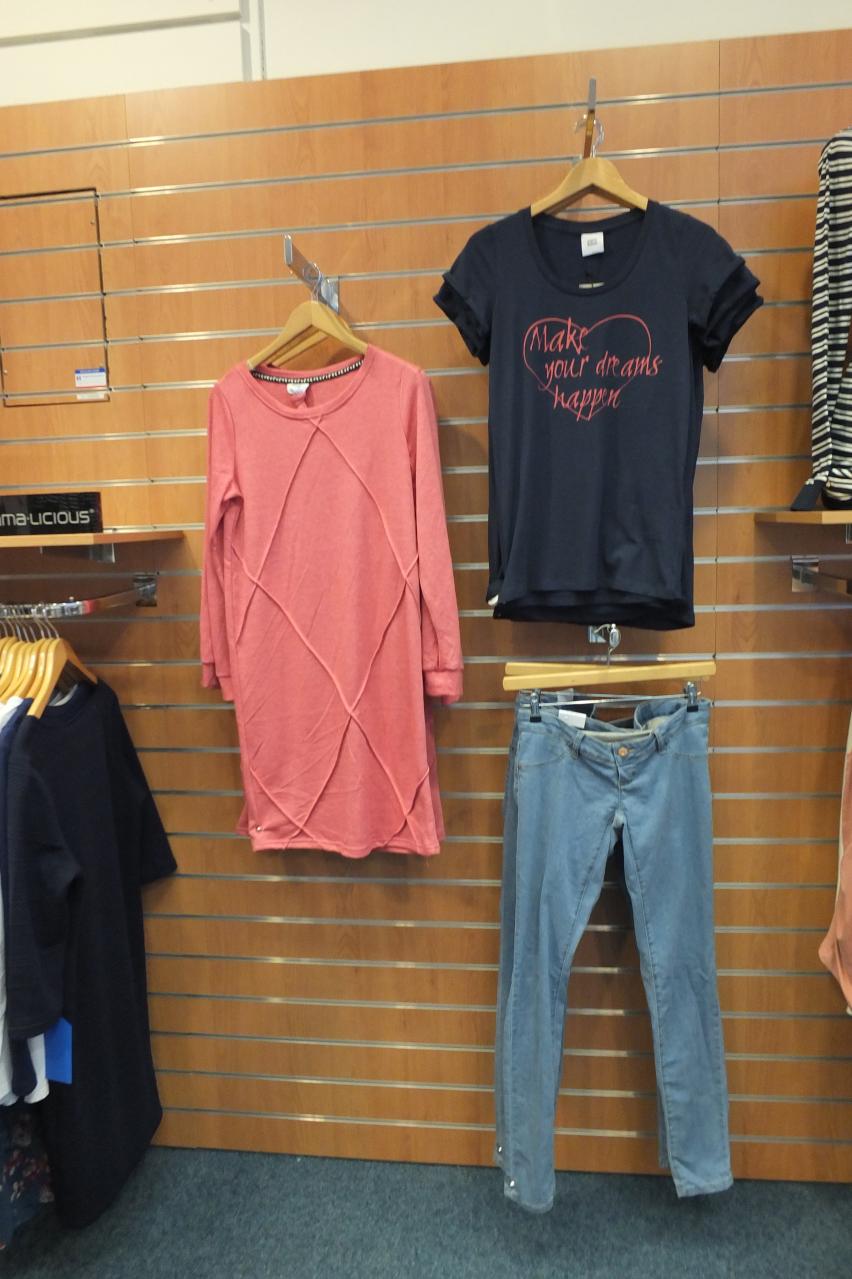This vertically oriented photograph depicts the interior of a women's clothing store with a wooden tan-colored wall adorned with horizontal metal bars used to hang garments. The central focus is on three articles of clothing: a pair of jeans, a black t-shirt emblazoned with a pink heart and the inspirational phrase "Make Your Dreams Happen," and a pink sweater or blouse. These items are showcased prominently on hangers suspended from the metal bars. To the left, there is a lower rack of additional clothing items, primarily black shirts, with a small shelf above displaying a sign that partially reads "malicious." The right side of the image also reveals more clothing items, while the floor is covered in blue carpet. There are no visible price tags or store workers in the scene, and other clothes in the background are too distant to identify clearly.